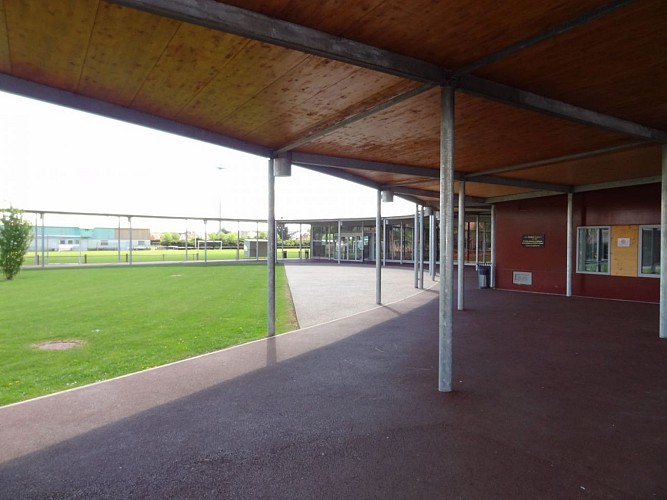The image depicts a daytime scene, likely taken around noon, focused on an exterior area that seems to be part of an educational or public facility. Dominating the right side of the image is a single-story building with reddish-brown walls and a distinctive wooden roof supported by silver metal pillars, which extends outward and around the structure. At the front, there is a rectangular window set into the wall, flanked by a notable yellow area. The left side of the image features a well-manicured grass field with a single tree growing prominently. The background reveals additional buildings, including some light blue and beige structures, as well as a vast open field that possibly contains a soccer net. The ambient light is very bright, casting minimal shadows, and coloring the sky a near white with no visible clouds. The colors throughout the scene include dark red, brown, gray, green, blue, and red, with most of the grass situated towards the left and the primary building focused on the right. The image overall doesn't contain any text.